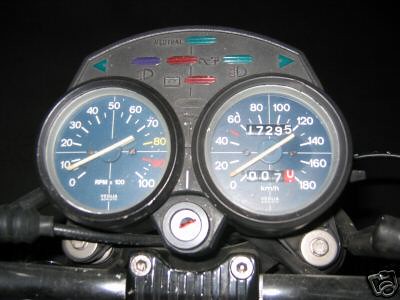The image showcases the control panel of a motorcycle, featuring detailed dials and meters. The prominent dials include the RPM gauge, currently indicating 10 RPM, and the speedometer, which reads approximately 10 miles per hour. The face of the dials is black with white numerals and markings. The RPM gauge is marked incrementally from 0 to 100, with additional markings at each five-unit interval. The speedometer, which also includes a kilometer per hour scale, displays speeds up to 180, with increments of 20 and additional markings for each five-unit interval.

Also visible are the odometer and trip meter. The odometer shows the motorcycle has traveled 17,295 miles, while the trip meter indicates a recent journey of 7 miles. Surrounding the dials are several indicator lights, including turn signals, headlights, and emergency flashers, although one light's specific function is indistinguishable.

The image also provides a view of the motorcycle's handlebars, with the horn situated centrally. Various bolts and fixtures that secure the handlebars are visible, underscoring the detailed mechanics of the motorcycle's control system.